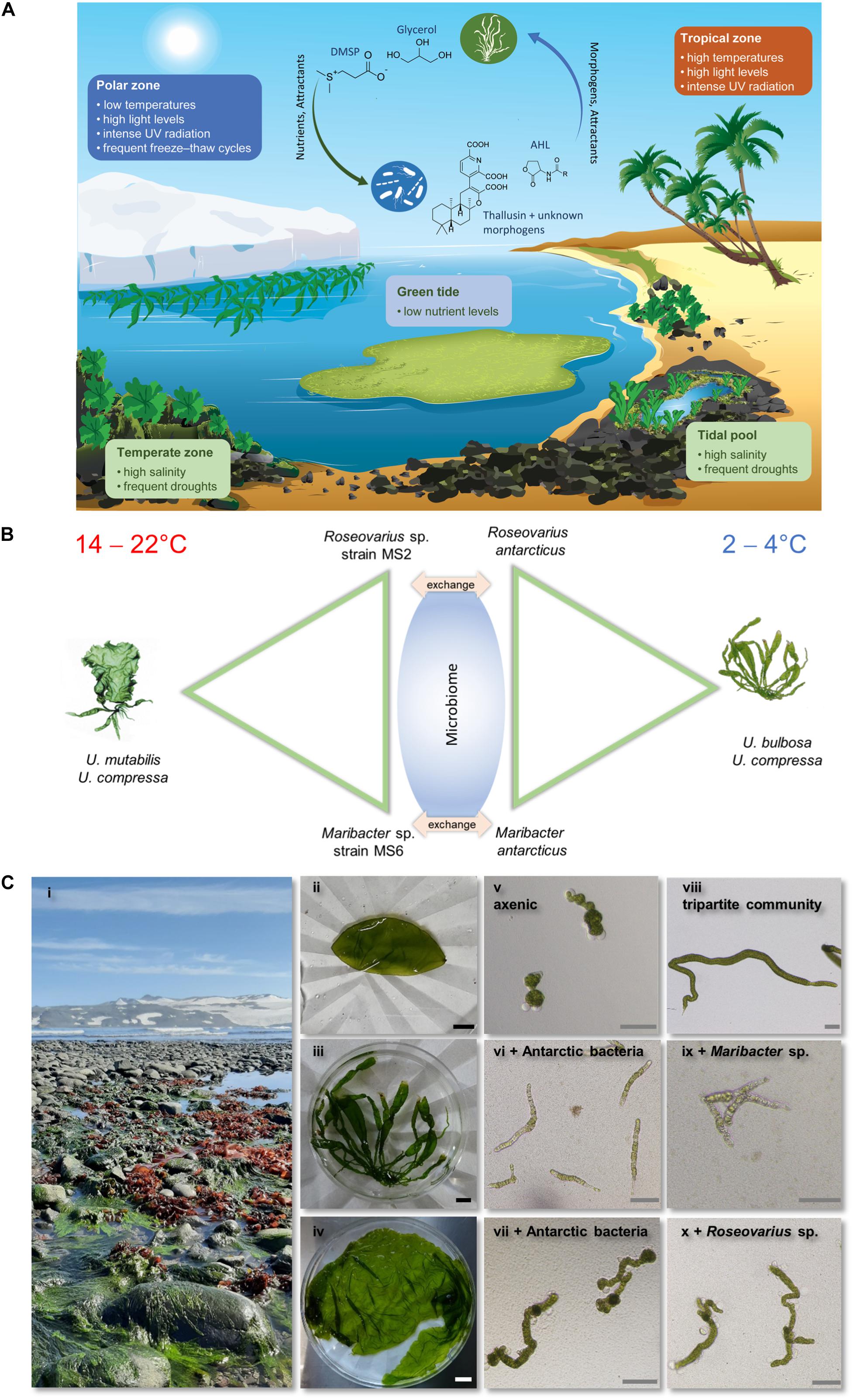This vertical, rectangular instructional image is divided into three distinct sections labeled A, B, and C. At the top, section A features a detailed drawing of a beach alongside a body of water, with various zones clearly labeled: Polar Zone, Tropical Zone, Tidal Pool, and Temperature Zone. Small rectangles with rounded corners containing text explain the elements within the illustration. The middle section, B, presents a diagram labeled "Microbiome" with the word "Exchange" positioned above it. This part shows symmetrically arranged arrows pointing left and right to two green plant segments. 

Section C at the bottom is composed of ten smaller segments that mainly display different types of fungi and bacteria. The leftmost image provides a broad overview of rocks covered in moss, while the nine subsequent segments offer close-up views of various bacterial and moss specimens. This part resembles a data table, providing detailed insights into the specimens found in the beach ecosystem. Overall, the layout systematically educates viewers on coastal habitats and microbial life through clearly segmented, informative visuals.